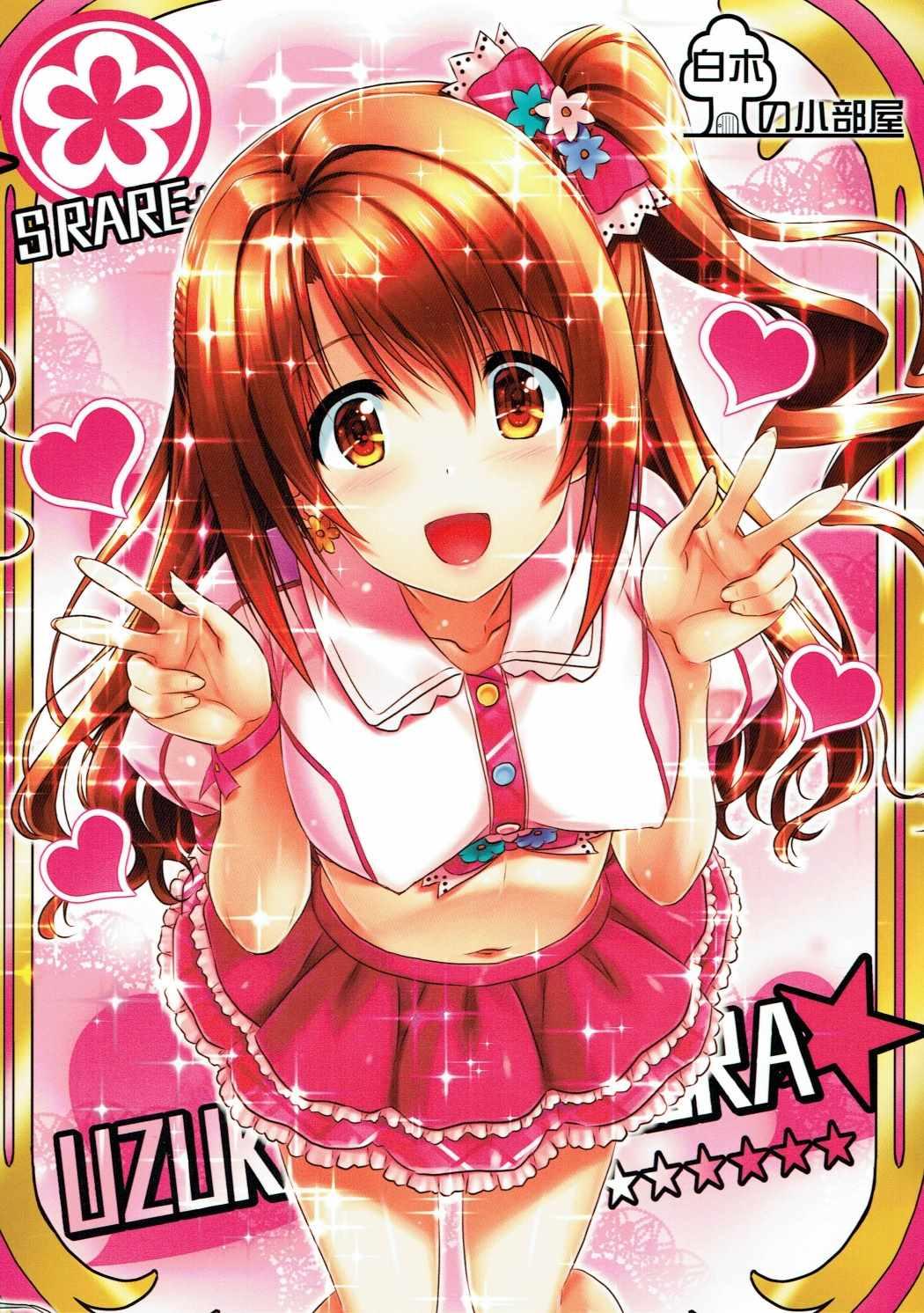This anime poster features a teenage girl standing in the center against a vibrant, pink, and sparkly background adorned with heart shapes and various designs. The background has gold edging, particularly visible on the sides, with a flower design on the top left corner accompanied by the text "S-R-A-R-E", and some Japanese characters in the top right corner. Below the character, the name "UZUKU ARA" is written, followed by six stars.

The character has long, reddish-brown hair that sparkles, and large golden-brown eyes. She is smiling directly at the camera while making a peace sign with both hands. She wears a short, light pink shirt with a darker pink strip down the front, adorned with multicolored buttons, exposing her midriff. Her skirt is extremely short, hot pink with a two-layered frill, where the frills are pale pink, almost white, and decorated with some bling around the edges. On her right wrist, she wears a pink wristband. The scene is filled with additional pink hearts and white stars, creating a lively and cheerful ambiance.